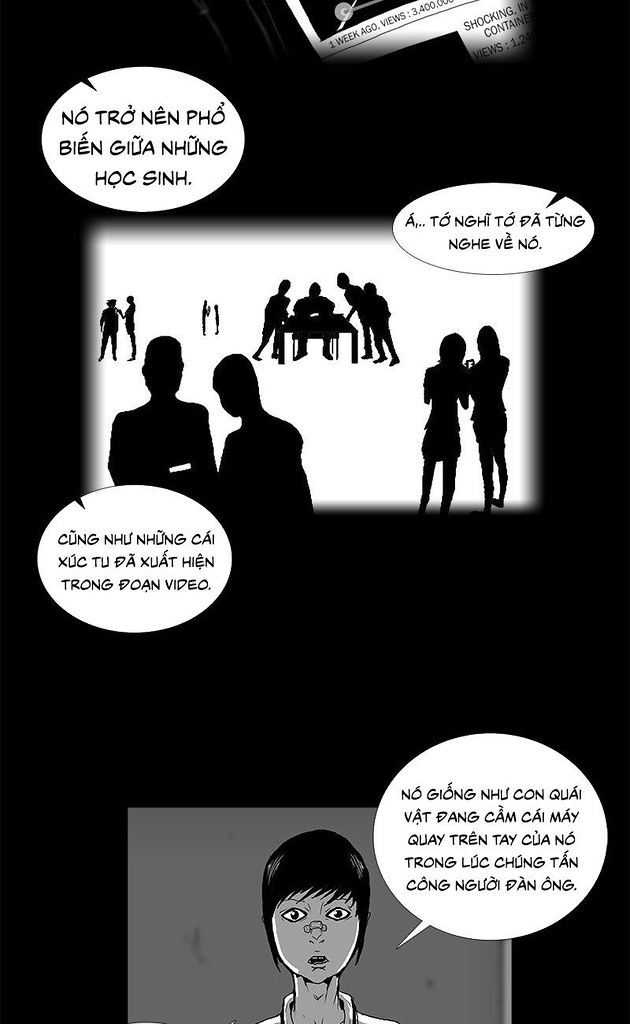A Vietnamese comic strip featuring two distinct panels: The first panel, in stark black and white, depicts silhouettes of people gathered in a room. Some figures are standing while others sit around a table, suggesting a meeting or discussion. Four text bubbles in Vietnamese are scattered around this scene, enhancing the mystery. The second panel focuses on a young woman with short black hair and an expression of surprise. A band-aid crosses her nose, and her wide eyes add to the sense of intrigue. This panel also contains a lengthy Vietnamese speech bubble, hinting at a significant dialogue moment connected to the earlier scene. The overall aesthetic is minimalist yet enigmatic, drawing the viewer into the story through its contrasting use of light and shadows.